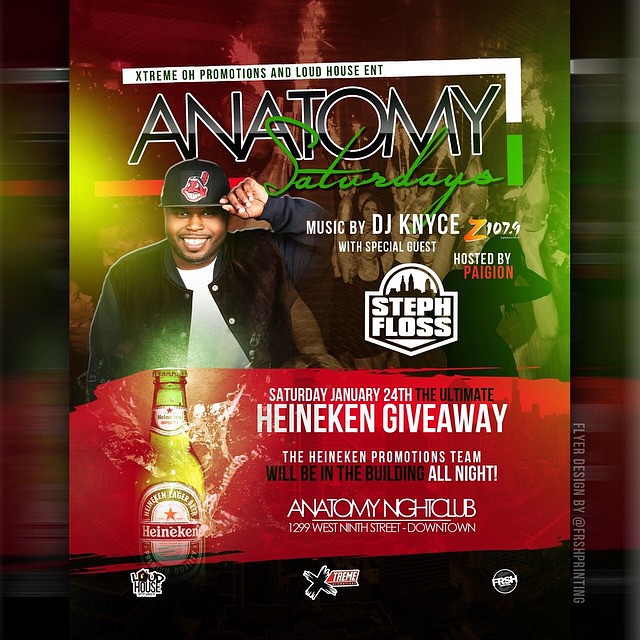This vibrant promotional flyer for Anatomy Nightclub's "Anatomy Saturdays" on January 24th is a rich blend of photography and graphic design elements. Prominently featured is DJ Nice KNYCE, an African American man donning a black jacket, white t-shirt, and a Cleveland Indians cap, smiling confidently with his left hand on the brim of his cap. The event, jointly presented by Extreme O Promotions and Loud Noise Entertainment, boasts special guest Steph Floss from Z1079, and is hosted by Paigion. The flyer, enhanced with a blurred background of clubgoers under green and red lighting, highlights the Ultimate Heineken Giveaway, with the Heineken Promotions team present all night. Detailed information about the event, along with logos and a dynamic Heineken bottle with a red paintbrush stripe, add to the appeal at the bottom of the flyer.